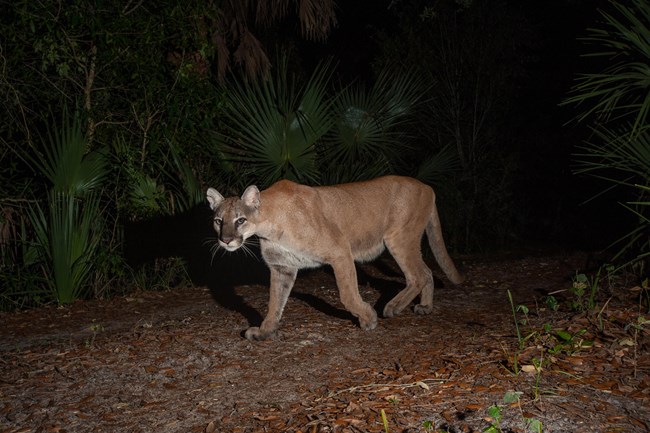Set against a shadowy jungle backdrop with dense foliage and large fronds, this nighttime photograph reveals a stunning wild cat, likely a jaguar or puma, captured by a trail camera. Illuminated in the center, the cat's powerful and sleek body is on display with a coat of pale, yellowish-tan fur, dark brown on its face and nose, and a striking white and grey patch on its chest. In mid-stride, the feline's muscular form and long, low-hanging tail are evident, as are its large ears and prominent whiskers. The creature's steady gaze, directed straight at the camera, gives an impression of eerie awareness. The surrounding ground is a mix of mulch and scattered grass, typical of a woodland scrubland. The cat's shadow melds intriguingly with the soil and flora, enhancing the sense of its presence in its natural habitat.